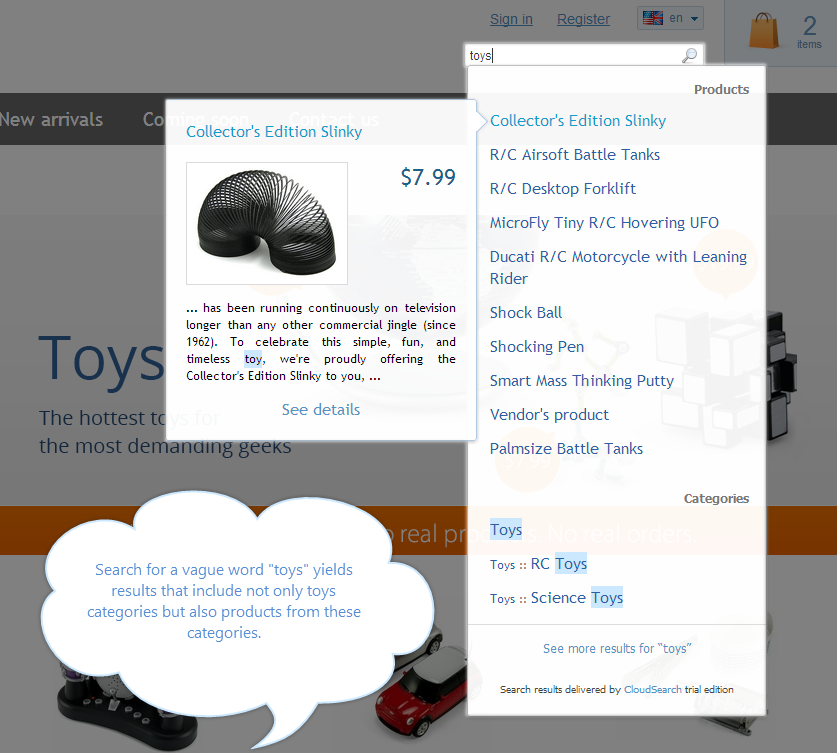The webpage in the image showcases an online shopping site specializing in toys. On the left side of the page, there is a prominently featured section for the "Collector's Edition Slinky," enclosed in a square. Below the bold header is an image of a Slinky priced at $7.99. Accompanying the image is a description celebrating the Slinky's enduring legacy: "Has been running continuously on television longer than any other commercial jingle since 1962. To celebrate the simple fun and timeless toy, we're proudly offering the Collector's Edition Slinky to you. See details."

On the right side of the webpage, a pop-up window is present. At the top of this pop-up, there is a header labeled "Products." Below this header, the "Collector's Edition Slinky" is highlighted, emphasizing its selection. The pop-up continues with a list of other products: "RC Airsoft Battle Tanks, RC Desktop Forklift, Microfly Tiny RC Hovering UFO, Ducati RC Motorcycle with Leaning Riders, Shock Ball, Shocking Pen, Smart Mask Thinking Putty, Vendor's Product, Palm Size Battle Tanks."

Further down, the pop-up displays the "Categories" section, listing: "Toys, Toys, RC Toys, and Toys, Science Toys." To the left of this list, a speech bubble contains the text: "Search for a vague word, 'toys', yields results that include not only toys categories, but also products from these categories."

The main background of the page seems to be a general toy section, but it is obscured by the pop-up, making it difficult to see the detailed layout of the webpage itself.